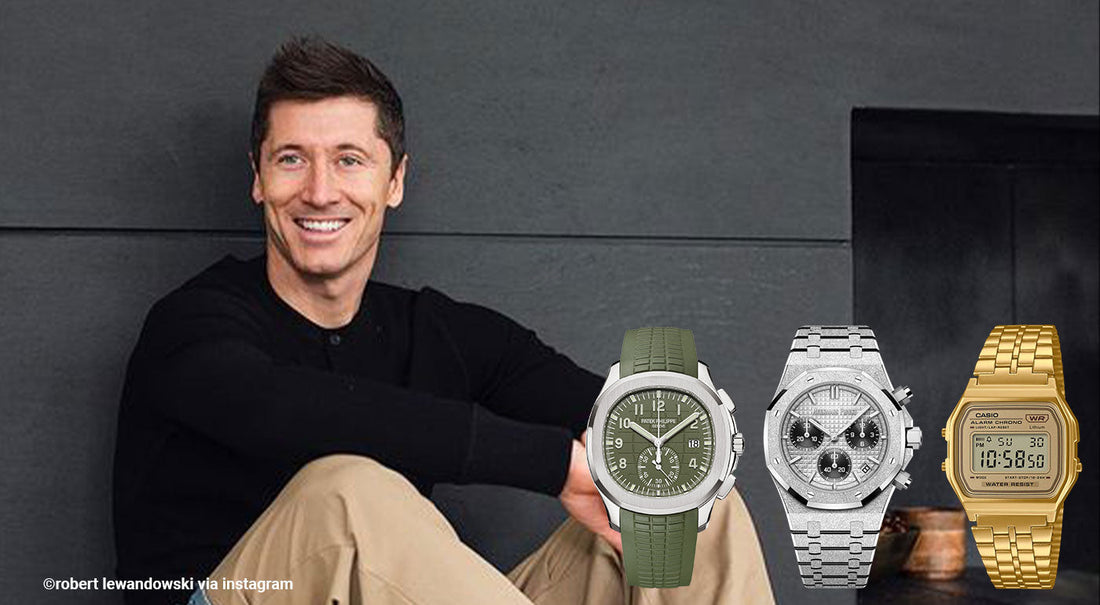The image features a smiling man with a light complexion and short, dark brown hair, which is styled into a neat wave at the front. He is dressed in a black long-sleeve thermal shirt, buttoned up, and a pair of brown khakis, seated comfortably with his hands resting on his knees. The man, identified by a small copyright text in the bottom corner as Robert Lewandowski via Instagram, is looking slightly off-camera, emanating a clean-cut and approachable demeanor.

The background is a dark gray wall, giving the photo a sleek and minimalist feel, suitable for an advertisement. In the bottom right corner of the image, three superimposed watch images are prominently displayed, each oriented with their faces towards the viewer. 

- The first watch features a green rubber band with a traditional clock face.
- The second watch boasts a metallic silver band with a chrome overlay and smaller black dials inside.
- The third watch is adorned with a gold band and a digital display reading "10:58:50."

These watches appear high-end and professionally presented, reinforcing the impression that this is an advertisement, possibly for a luxury watch brand. The overall composition, highlighting both Robert Lewandowski and the watches, suggests a modern, stylish aesthetic.